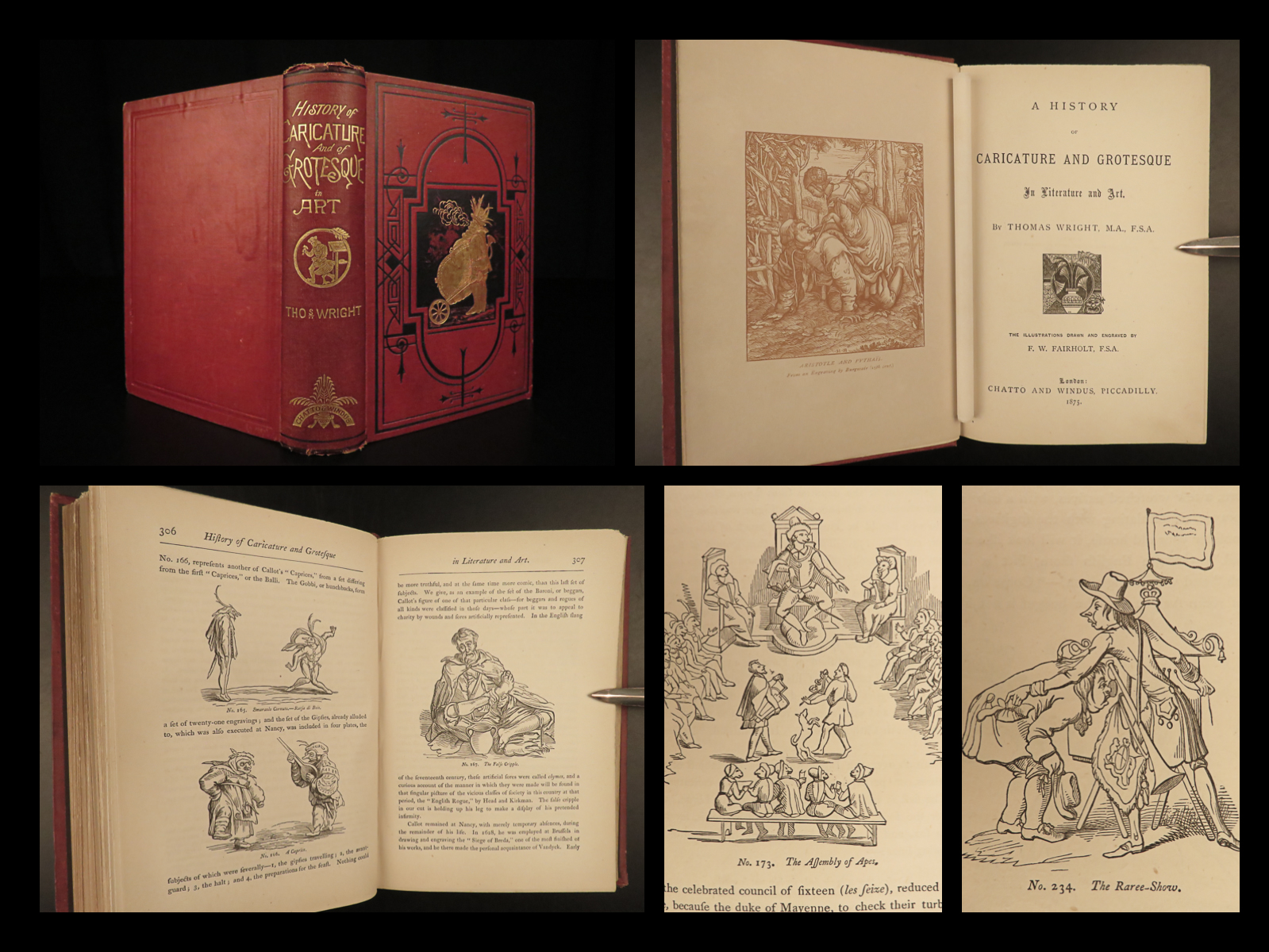The image features a collage of four photographs showcasing an antique book titled *The History of Caricature and Grotesque in Art*, set against a black background. 

At the top left, the book’s red cover and back are displayed. The front cover features an intricate gold design with black outlines, depicting a man pushing a wheelbarrow, while the title is embossed in gold along the edge. 

The top right photo reveals the book open to the title page, showcasing a detailed wood carving of a man holding a deceased lady. The title, *The History of Caricature and Grotesque in Art*, is prominently displayed in gold lettering.

The bottom left image shows the book opened to the middle, presenting pages adorned with small illustrations and text, including a depiction of a man bent over and various other figures, though the text is partly unreadable.

In the bottom right photograph, a closer look at more illustrations is provided. One page shows a king seated on a throne surrounded by servants, and the opposite page depicts a man in a jacket carrying a horn with another figure bowing beneath him, suggesting a theme set in the Middle Ages or the late 17th century. A pen is casually placed, pointing toward one of the pages, adding a modern touch to the historic visual elements.